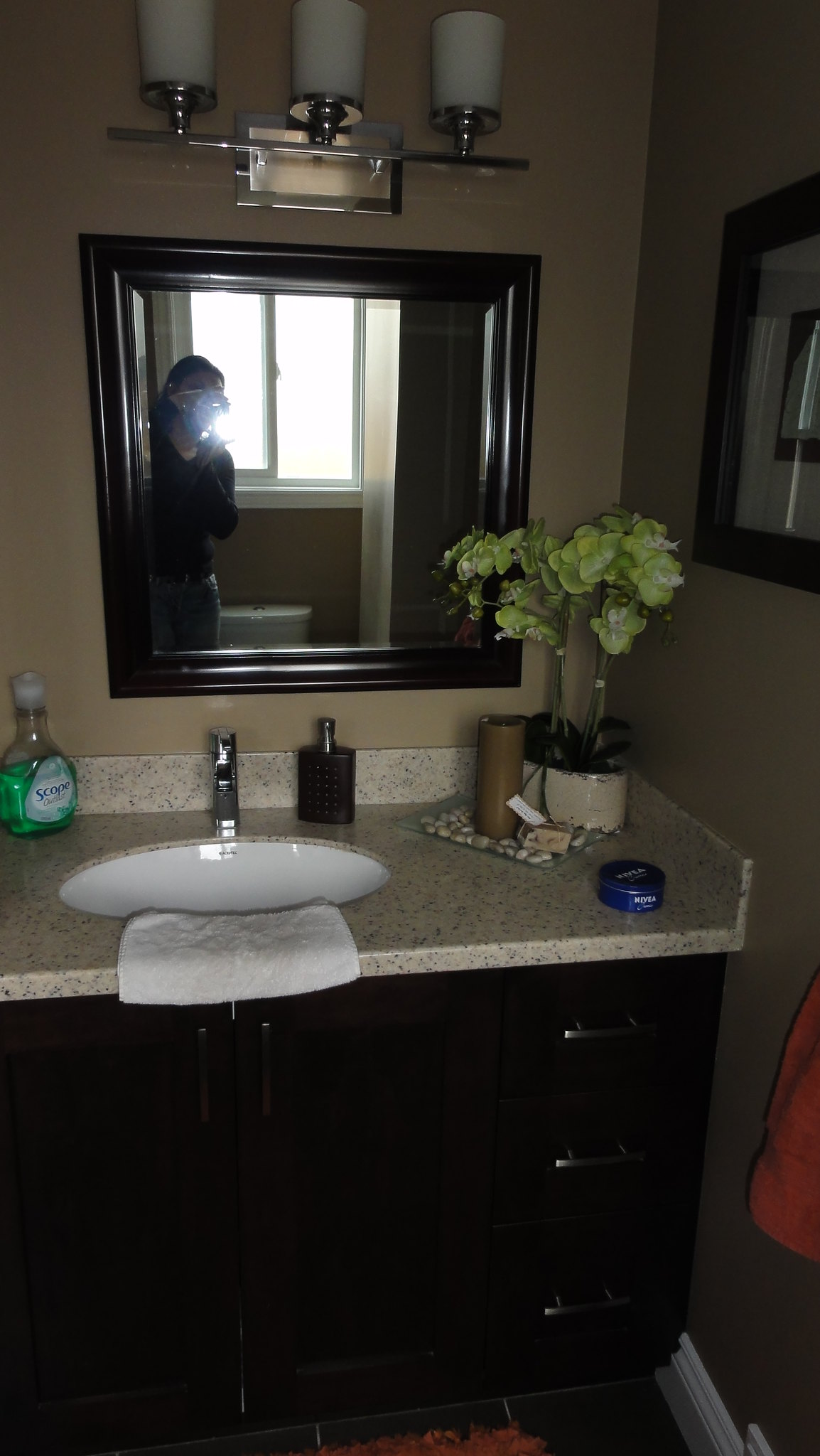The image features a stylish bathroom with a single white sink set in a sophisticated granite-style countertop. The countertop has a warm brown background adorned with black speckles, creating a textured and luxurious look. A sleek silver faucet complements the sink, while a neatly folded white washcloth rests in front of it. To the left of the sink, a bronze-colored, square soap dispenser with a pewter pump adds a touch of elegance. Adjacent to the soap dispenser, a gray display dish holds an arrangement of brown rocks, offering a natural and calming element.

Further enhancing the aesthetic, there is a brown pillar candle adding a cozy ambiance. In the corner of the countertop stands a delicate flower arrangement that resembles an orchid, featuring yellow and white blooms with a long stem and green flowers at the base. It's unclear whether the flowers are real or artificial, but they certainly bring a refreshing touch of nature indoors. Beside the flowers, there is a mysterious blue canister, slightly larger than a typical chewing tobacco container, adding an element of curiosity.

The cabinetry below the sink is crafted from very dark brown wood, providing a rich contrast to the lighter elements and tying the entire bathroom decor together seamlessly.